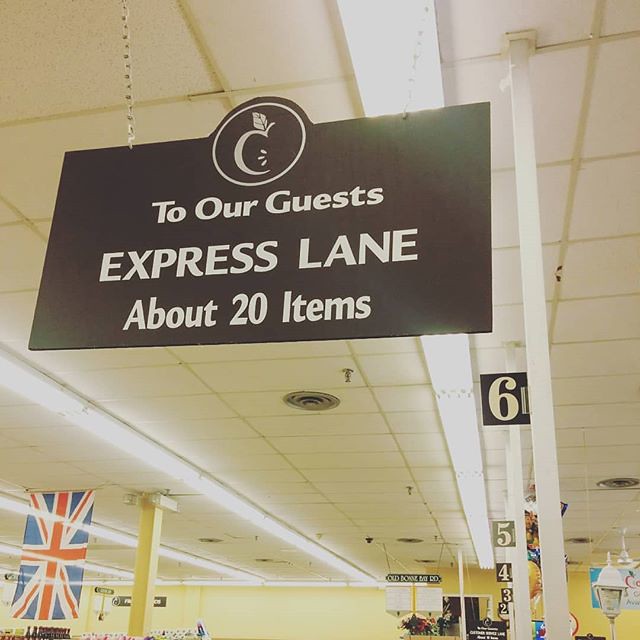The image is a professionally-taken square color photograph of the interior of a supermarket, captured from a low angle in the checkout lane area. The main focus is on a large black hanging sign in the upper center portion, which reads in white text: "To Our Guests, Express Lane, About 20 Items." Above the text is a logo featuring a half-eaten apple with a leaf, likely representing the supermarket’s brand. The ceiling, visible due to the upward angle, is white with a square tile design and lined with long fluorescent lights that illuminate the space. Multiple checkout lanes are visible, marked by poles with black frames and white numbers, specifically lane six in the forefront. The background reveals lanes five through two, offering a perspective that extends deep into the store. A yellow wall and a uniquely placed British flag hanging from the ceiling add distinct elements to the setting, suggesting the supermarket is possibly located in Britain. Overall, the image conveys a well-lit, organized grocery store aisle, with all elements sharply exposed, suitable for a magazine feature.